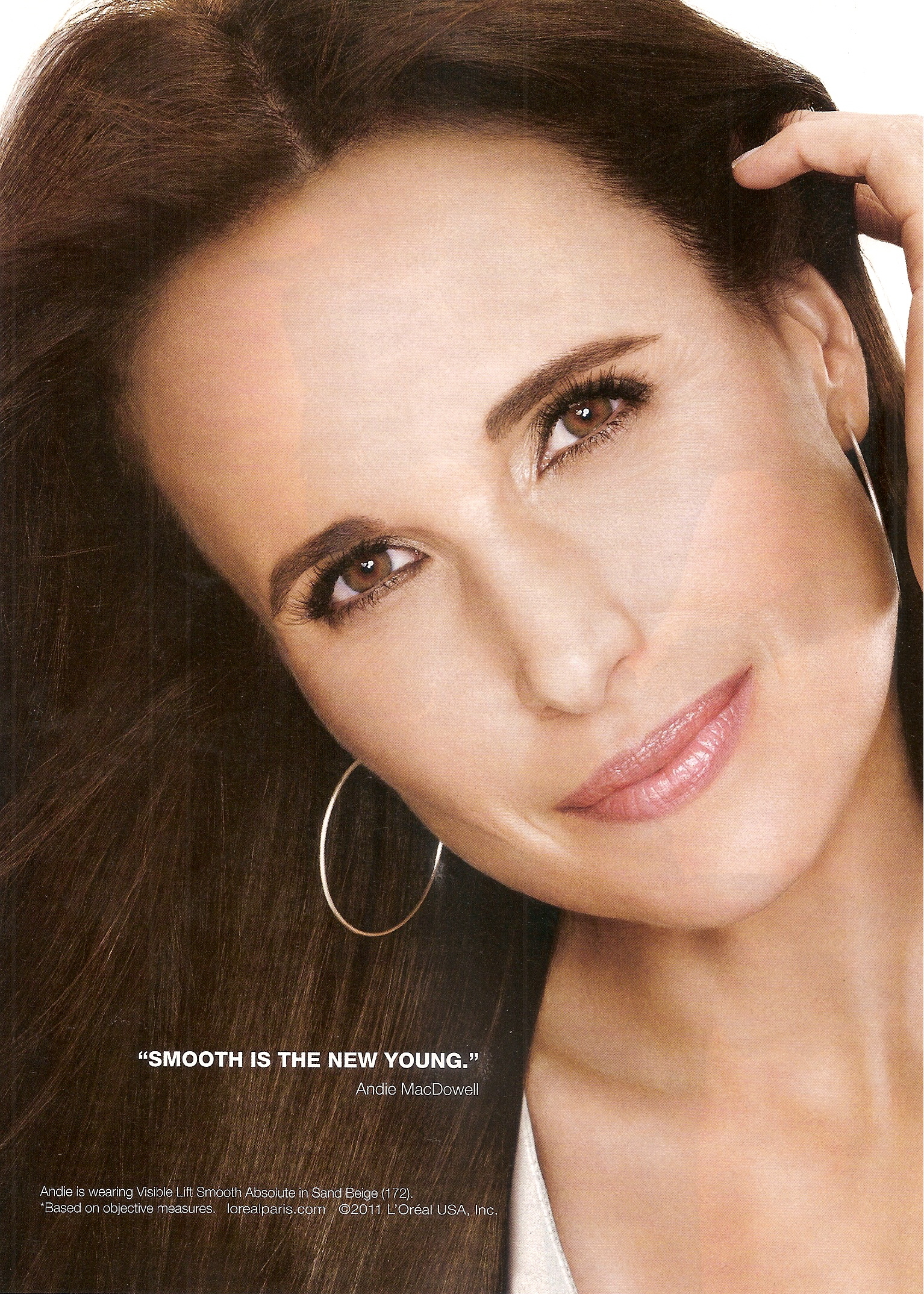This advertisement features a close-up image of the actress and model Andy McDowell, known for her role in "Groundhog Day." The photo, slightly grainy with a vertical texture, shows Andy in a white top, possibly a tank or scoop shirt, and silver hoop earrings in each ear. Her long, dark brown hair is styled over her right shoulder, with her head tilted to her right. She has brown eyes, black eyebrows, and is wearing light pink lipstick with a serious, neutral expression. The backdrop of the photo is white, emphasizing the text overlay which reads, "Smooth is the new young Andy McDowell." Smaller, barely legible copyright information is present below the main text, hinting at affiliation with L'Oreal makeup products.